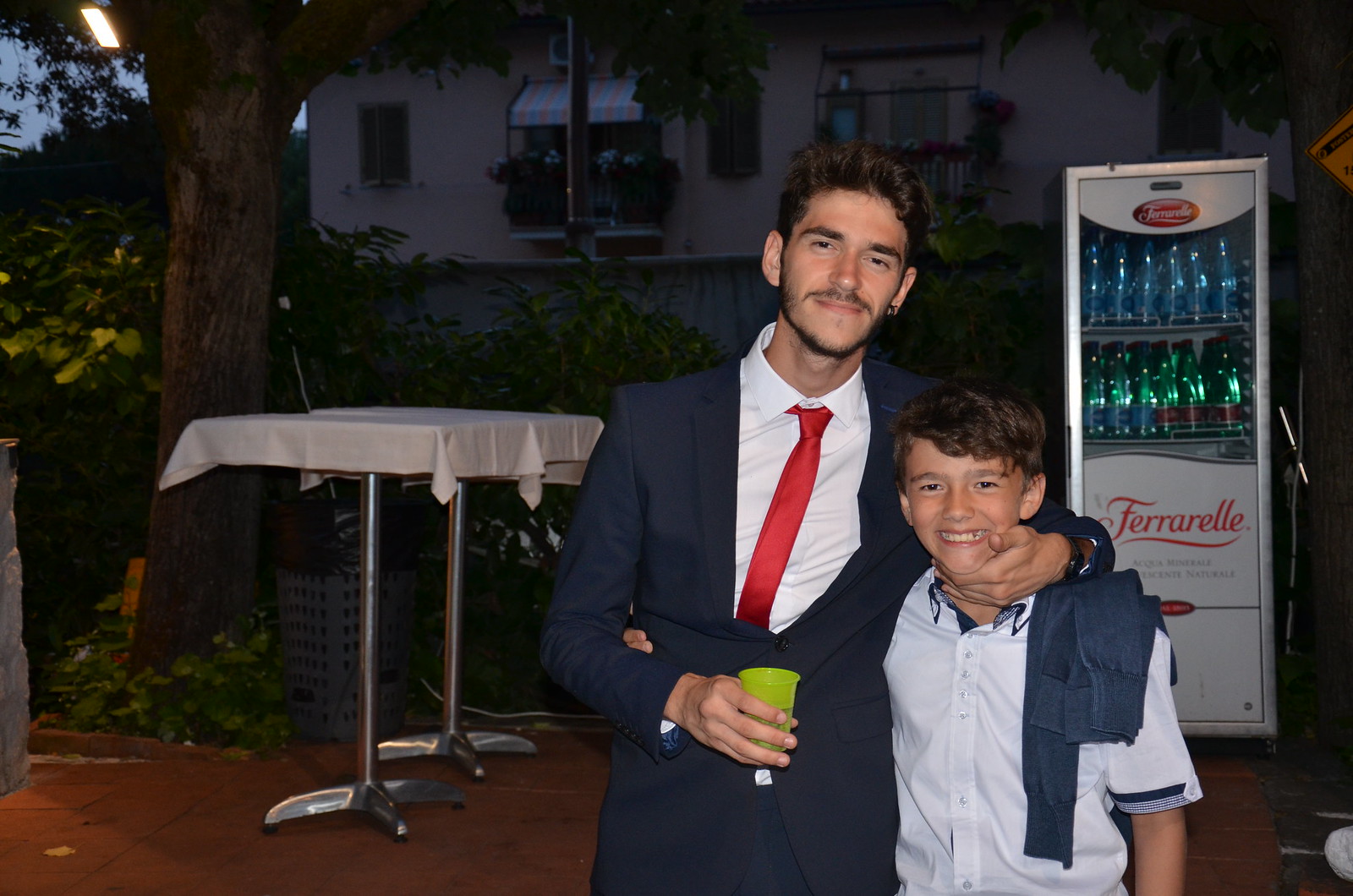In the photograph, an older man, possibly in his late teens to mid-twenties, stands closely with a young boy who looks around nine to eleven years old. They both appear Caucasian with brown hair, and they are smiling warmly, suggesting they could be related, perhaps a father and son or older and younger brothers. The older man is dressed in a navy suit with a red tie over a button-down shirt, his hair is well-styled, and he sports facial hair and an earring. He has his arm around the boy’s shoulder, signifying a close bond. The boy looks happy, mirroring the older man's expression.

They are outdoors, possibly at a European cafe setting. The scene is set against the backdrop of an apartment building with a fence in front of it. It's either night-time or approaching it, signaled by a hanging light from a tree on the left side of the image. The ground is comprised of dark wooden or red patio stones. Around them are high stool-sized tables with metal bases and white tablecloths, suggesting a celebratory or casual gathering. To the right, there is a silver vending machine labeled 'Ferrarelle', likely a sparkling or mineral water brand. In addition, bushes and a tree are visible on the patio, adding to the ambiance of the evening setting.